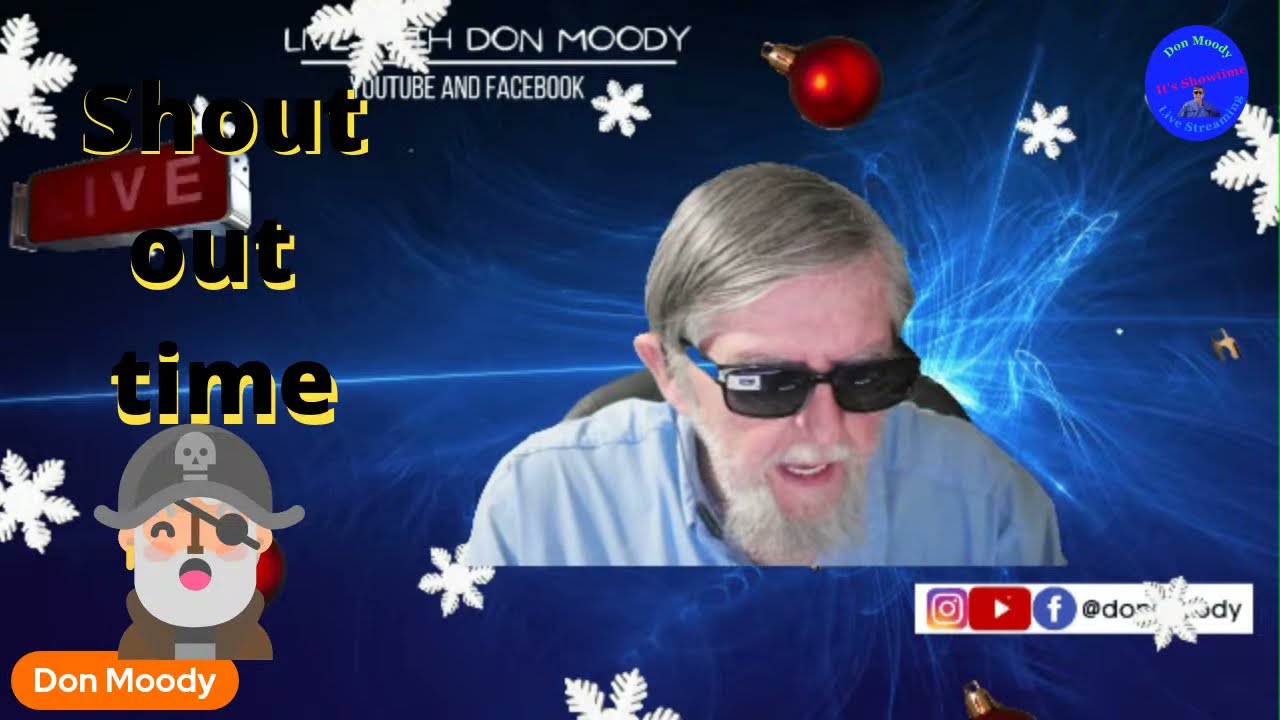In the center of the image, a man with blonde hair, a white beard, and large sunglasses gazes downward while seated. He wears a blue t-shirt and is positioned against a deep navy-blue background adorned with snowflake patterns. White light glows from multiple points, enhancing the scene. Above him, bold text reads "Live with Don Moody, YouTube and Facebook," while to the left, a clearly marked "Shout Out Time" banner is visible. Additionally, a small pirate illustration with a white beard and eyepatch appears in the bottom left corner. The pirate design is complemented by an orange background that reads "Don Moody" in white letters. Different social media icons for Instagram, YouTube, and Facebook are displayed prominently in the lower right corner near the phrase "@Don Moody." This image is rich with decorative elements and promotional details for Don Moody's social media presence.